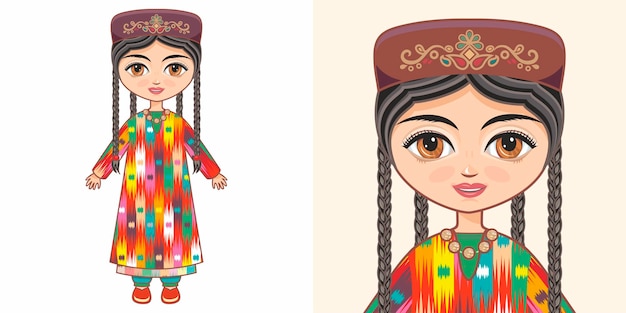The image consists of two side-by-side cartoon-style illustrations, presumably from a Nepalese or Eastern Slavic tradition. The left illustration showcases the full body of a cartoon doll or little girl, featuring exquisite details like four black braids, two in the front and two in the back, and a brown floral-decorated hat. The girl has large, expressive amber eyes, strong eyebrows, and a small pink mouth. She's dressed in a colorful, long-sleeved pullover dress that reaches nearly to her feet, adorned with vertical splotched stripes of rainbow hues including green, blue, yellow, pink, purple, and red. Underneath the dress, she's wearing green pants that only show at the ankles, and red shoes. A circle bead necklace adorns her neck.

The right illustration zooms in on the girl's face and shoulders, highlighting her detailed headpiece with floral and curlicue designs, large eyes, and intricate necklace. The background shifts from white in the full-body illustration to a slightly darker beige in the close-up. The intricate detailing and vibrant colors make the doll stand out in a striking and culturally rich portrayal.